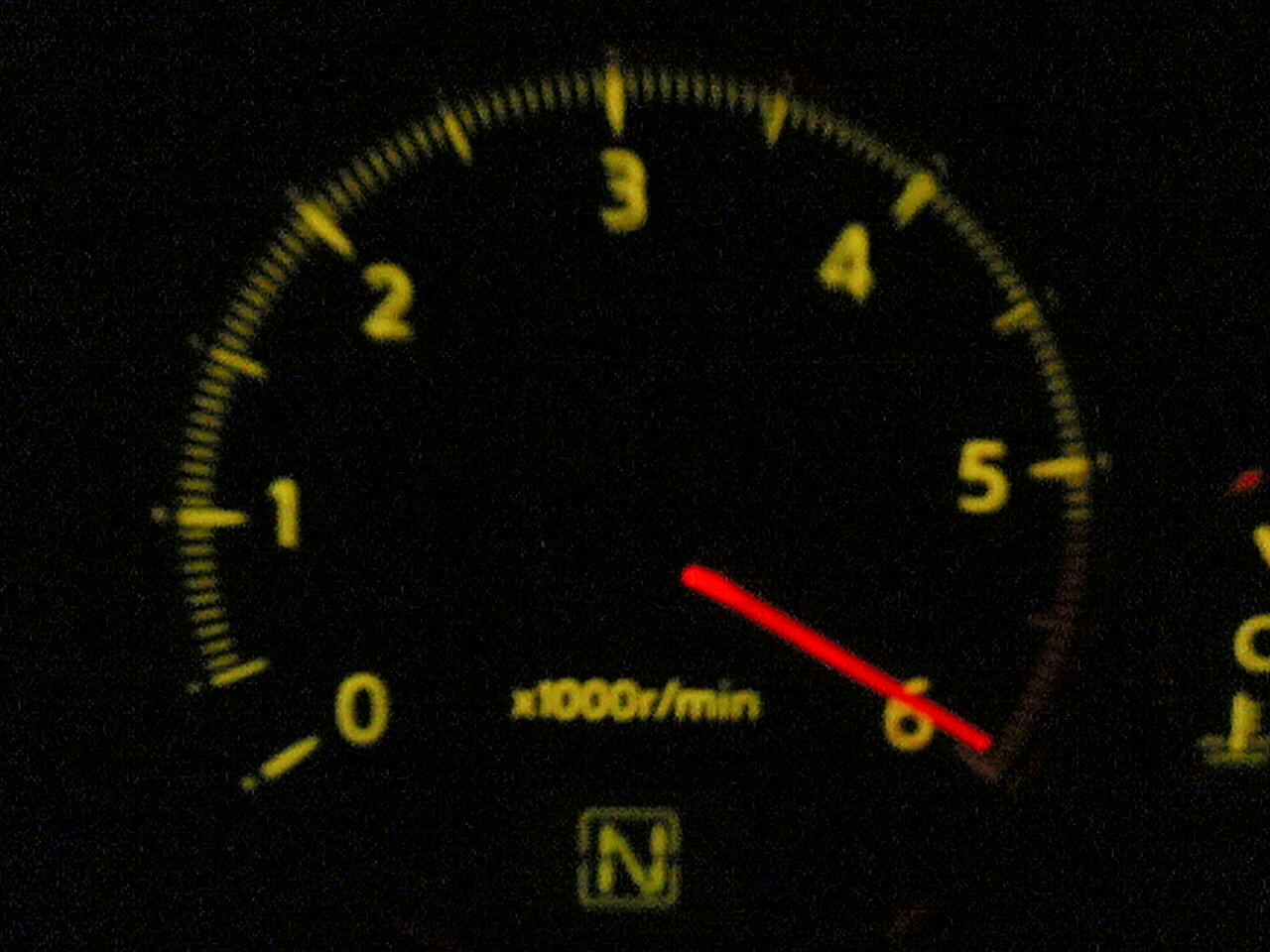Close-up image of a vehicle's tachometer displaying measurements in revolutions per minute (RPM). The tachometer's dial features yellow numbers ranging from 0 to 6, with incremental yellow lines between each main number. A prominent red needle indicates the current engine speed, pointing just before the 6 mark. At the bottom center of the dial is the label "X1000R-MIN," denoting the RPM measurement unit. Below this label, a yellow "N" and a yellow box are visible. The image is slightly blurry, but additional yellow text and a red mark can be seen to the right of the dial.